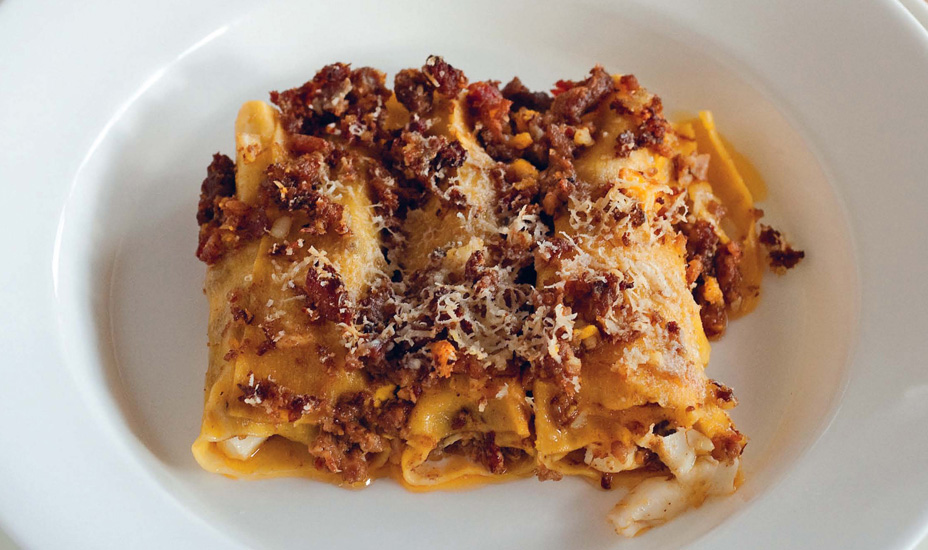The photograph, taken indoors, showcases a meticulously presented pasta dish in a white, shallow porcelain bowl set inside a slightly larger bowl. The dish features three large, rolled-up pasta noodles filled with what appears to be a white cheese, possibly mozzarella. Topped with finely grated parmesan cheese and crispy meat crumbles, likely a mix of bacon bits and Italian sausage, the pasta has an orange tinge, suggesting it was baked in a rich sauce. The noodles glisten under the light, hinting at a slight greasiness or oiliness to the presentation. Perfectly arranged and untouched, the dish looks clean and ready to eat, capturing a sense of both indulgence and careful preparation.